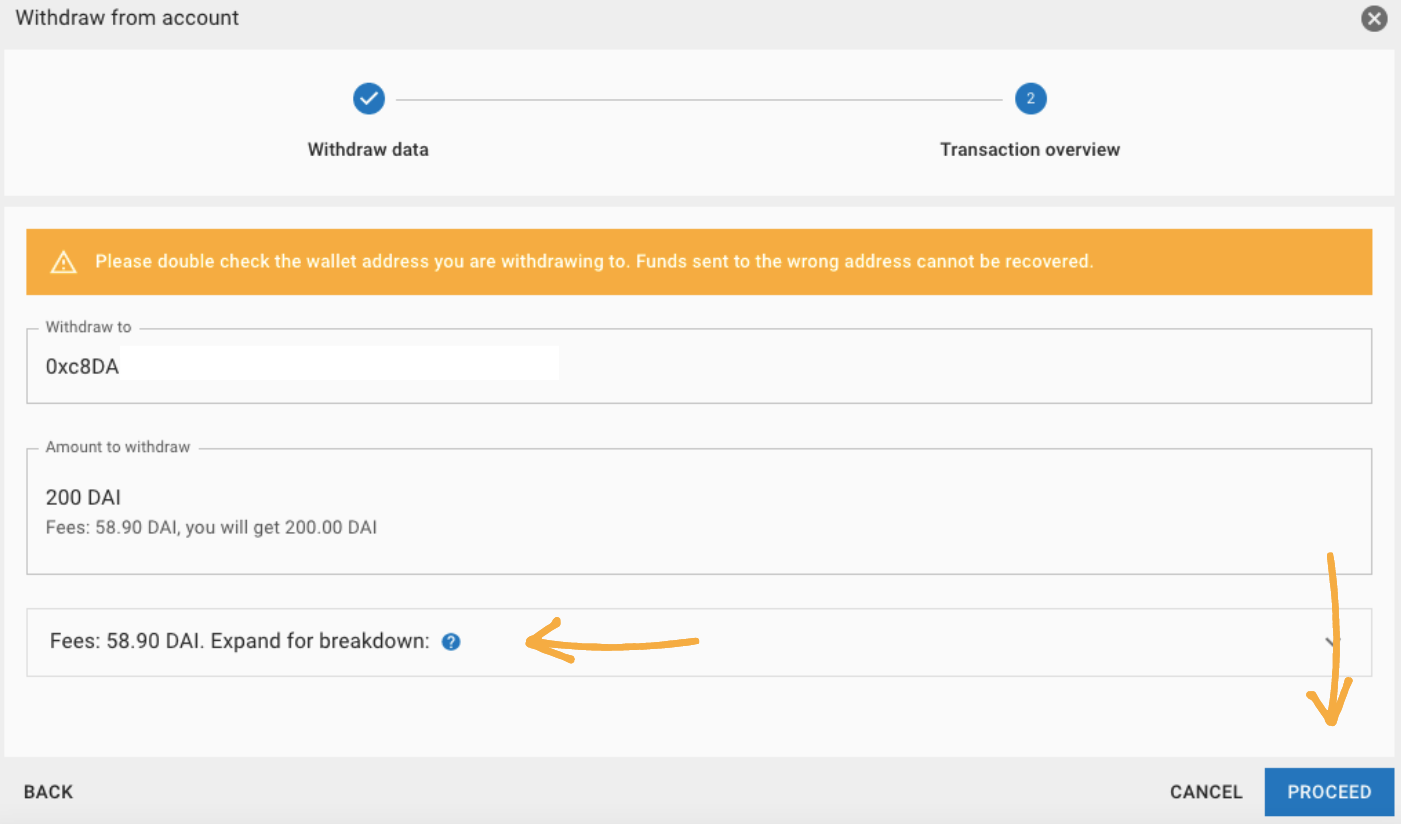The screenshot showcases an interface of a bank transaction process, specifically a cryptocurrency withdrawal. The sequence starts with a section titled "Withdraw from Account," marked with a blue check mark indicating this step is complete. The next step, "Transaction Overview," labeled as "2," has not been initiated yet.

An orange caution icon draws attention to an important notice, urging users to, "Please double check the wallet address you are withdrawing to. Funds sent to the wrong address cannot be recovered." This advisory emphasizes the critical necessity of verifying the recipient address multiple times to avoid irreversible errors.

Further details include:
- **Withdrawal Destination:** 0XC8DA
- **Amount to Withdraw:** 200 DAI (a cryptocurrency)
- **Fees:** 58.90 DAI

Accompanying these figures, an expandable option labeled "Fees breakdown" provides additional information. Hand-drawn arrows in orange highlight the "fees" section and the "proceed" button at the bottom of the interface, suggesting a focus on these areas.

At the bottom of the screen, there are navigational buttons, including:
- **Back**
- **Cancel**
- **Proceed** (highlighted in blue)

This comprehensive layout ensures users can review all necessary information before finalizing the transaction.